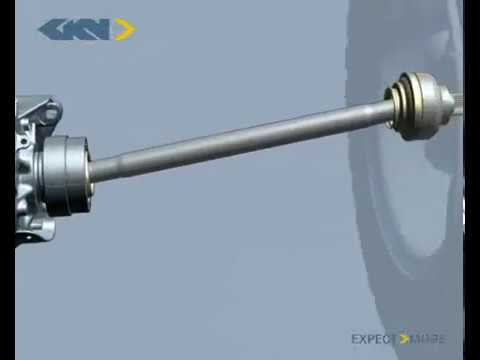The image appears to be a low-resolution computer-generated 3D illustration, likely a still from a video or graphic, showing a metallic mechanism that resembles an axle or driveshaft component possibly used in automotive applications. The primary feature is a long, gray steel rod extending at a slight angle across the image, supported by a larger, round base that is partially cut off at the edge. This rod may be related to hubcaps or lug nut removal, suggesting its use might be in vehicle maintenance or repair, potentially for large trucks. At the rod's visible end is a bulbous, rounded section, but details beyond this point are obscured. The background is uniformly gray, transitioning to a darker shade on the right. There are also some illegible markings at the bottom and some indiscernible, possibly blue letters at the top left. The entire image is framed in black on the left and right, adding to the sense that it's a segment from a digital screen.